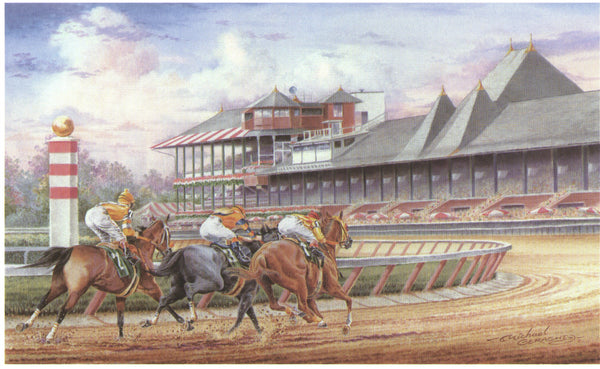This renaissance-style illustration depicts an intense horse race on a dirt track. Three jockeys, uniformed in orange caps, orange shirts, and white trousers, ride neck and neck, capturing the spirit of competition. The leftmost and rightmost jockeys are mounted on brown horses, with the jockey on the left in a more elevated riding stance, while the middle jockey rides a gray horse in a more hunched posture. All three horses are galloping at full speed, heading into a turn on the racetrack.

The racetrack itself is a rustic brown, surrounded by a vibrant scene of grandstands and medieval architecture. The grandstand, adorned with red sides and a gray roof, hosts an expectant crowd whose individual figures blur into the background. Strikingly, a red and white striped pillar topped with a golden sphere stands prominently on the left side, adding a regal touch to the scene. Beyond the track and grandstands lies a castle-like structure with gray roofs, golden tips, and red and white stripes, enhancing the historical ambiance.

The sky above is a dramatic blend of blue, purple, and red hues, dotted with clouds, suggesting a day rich with anticipation and excitement. The muted colors and detailed elements combine to create a vivid portrayal of a timeless sporting event.